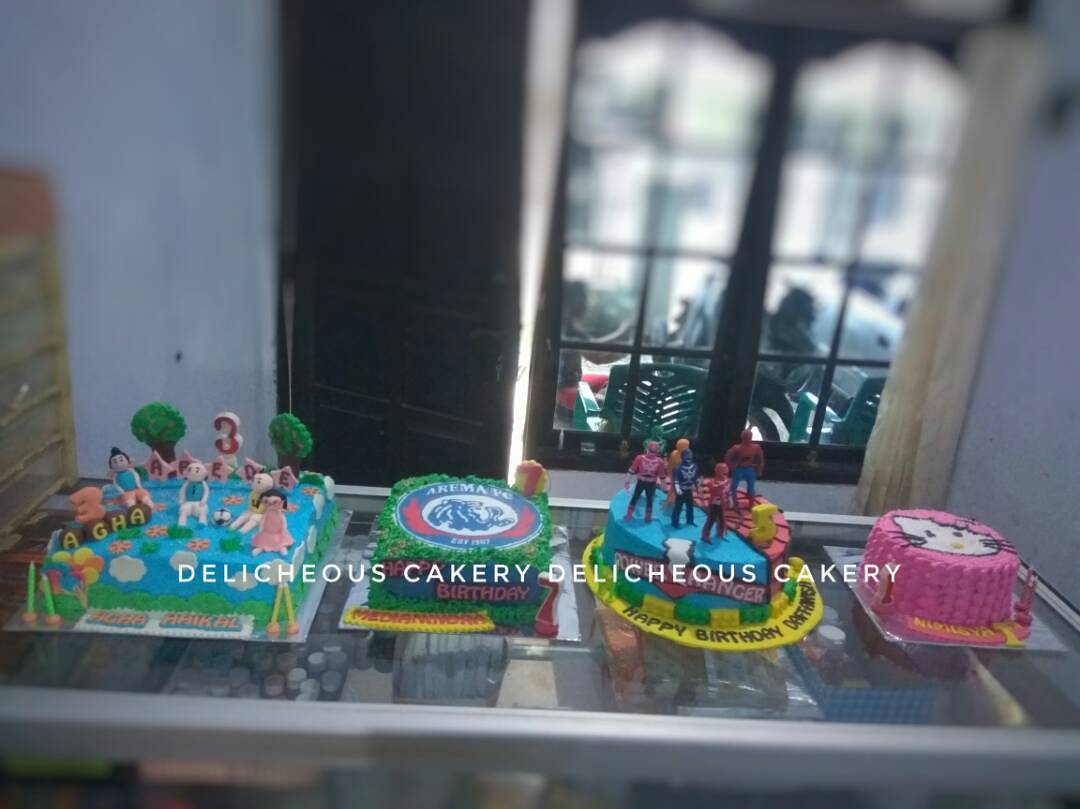In this detailed image of a cake shop counter, we see four intricately designed birthday cakes displayed on a glass display counter. Each cake is small but elaborate, placed from left to right. The first cake, themed with sky and grass motifs, features three little cartoon characters and is adorned with a number 3 candle, likely for a third birthday celebration. The second cake, green in color, bears a partially readable logo "AREMA" or "Aramans," along with a number 7 candle, suggesting it's for a seventh birthday. The third cake is a superhero-themed creation with prominent Spider-Man decorations and blurred candles, implying another third birthday. The final cake is a pink Hello Kitty design, crafted with exquisite detail. Superimposed across the bottom third of the image is the text "Delicious Cakery," albeit misspelled as "Delicheous Cakery," repeated four times. The background reveals a blurred scene featuring an open door and a window through which outdoor patio furniture is visible, indicating the setting is likely a café or restaurant. Wooden shelving is faintly visible on the left, and indistinct items are stored under the glass counter.